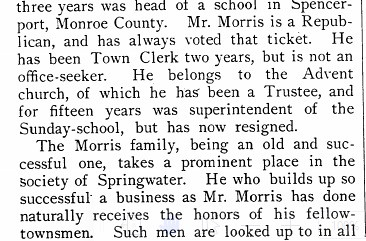The image depicts a cut-out paragraph from an old-fashioned, black-and-white newspaper or magazine article, set in a serif Garamond font on a white background. The text discusses Mr. Morris, a longstanding Republican who has consistently voted for his party. He served as the head of a school in Spencerport, Monroe County, for three years and has been the town clerk for two years, though he is not seeking office. Mr. Morris is a member of the Advent Church, where he was a trustee and superintendent of the Sunday School for 15 years before resigning. The Morris family is described as an old and successful family with a prominent place in the society of Springwater. Mr. Morris is recognized and honored by his fellow townsmen for building a successful business. There's a thin black line running vertically to the right of the paragraph, indicating a typical newspaper or magazine layout. The rest of the text is cut off, leaving the final sentence incomplete.